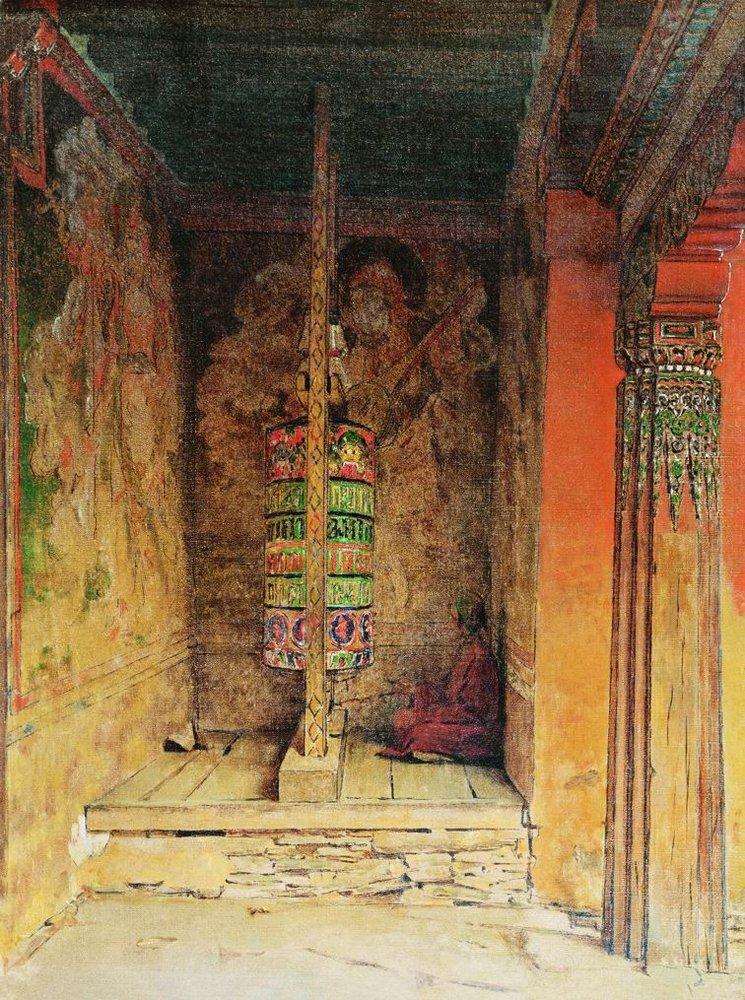This captivating painting showcases a richly colored scene filled with intricate details and figures. Dominated by hues of orange, yellow, red, green, brown, and black, the painting features a semi-outdoor setting that draws the viewer's eye to a central figure—a small person clad in a red robe, seated against a wall. This figure contrasts starkly with towering figures in the background, who are adorned in robes and nearly fill the entire canvas. The artwork depicts a sandy surface at the bottom leading to a step made of brick or concrete, which supports a wooden platform.

A central, striking element of the scene is a vibrant prayer wheel with six colorful segments, seemingly suspended in front of faded images that might include musicians and a mandolin player, their features blurred and rendered in muted tones of beige and brown. The right side of the painting reveals a stone pillar, transitioning from yellow at its base to a deep orange at the top, against a backdrop of wooden beams blackened by charcoal. The left side wall hosts an additional faded figure, adding more depth to the surroundings. Despite the dim lighting, the intricate drawings and implied narratives on both the walls and the prayer wheel draw viewers into an intriguing, historical atmosphere.